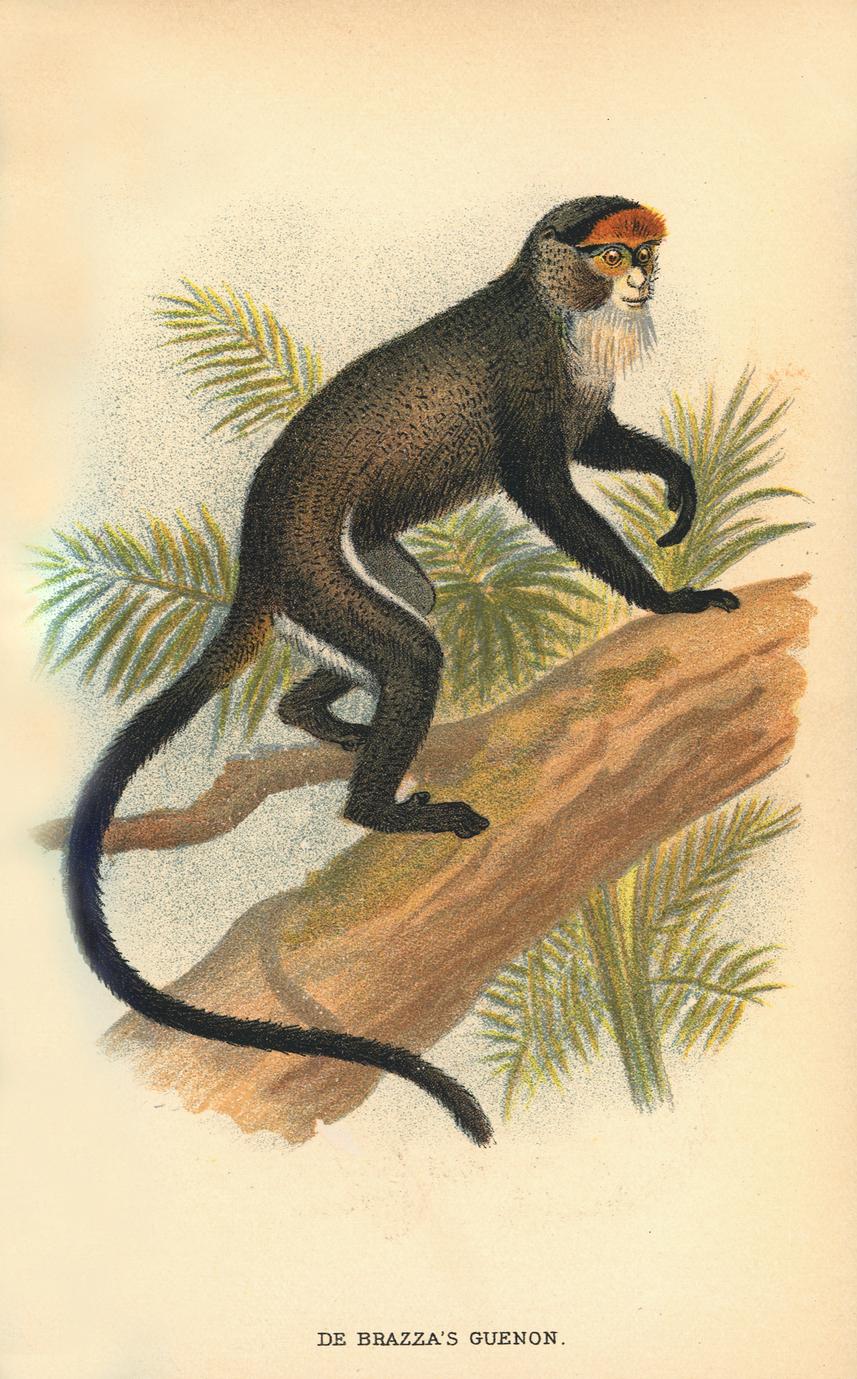The image depicts a detailed, colonial-style painting of a De Brazza's guenon, a type of primate. In portrait orientation, the monkey with a small, baboon-like face is characterized by its blackish-brown fur interspersed with brown, and it has distinctive features including a long white beard and a red, light orange crown or cap around its face. The nimble guenon, featuring long arms, legs, and a remarkably long black tail that wraps around a wide tree branch, climbs or rests on it. The background showcases large palm fronds and ferns against a mingled light pink or beige backdrop, with patches of blue around the ferns, contributing to the etching- or engraving-like quality of the image. The monkey is oriented looking off to the right from the viewer's perspective. The painting is detailed enough to list the name "De Brazza's guenon" at the bottom, highlighting the subject's identity.